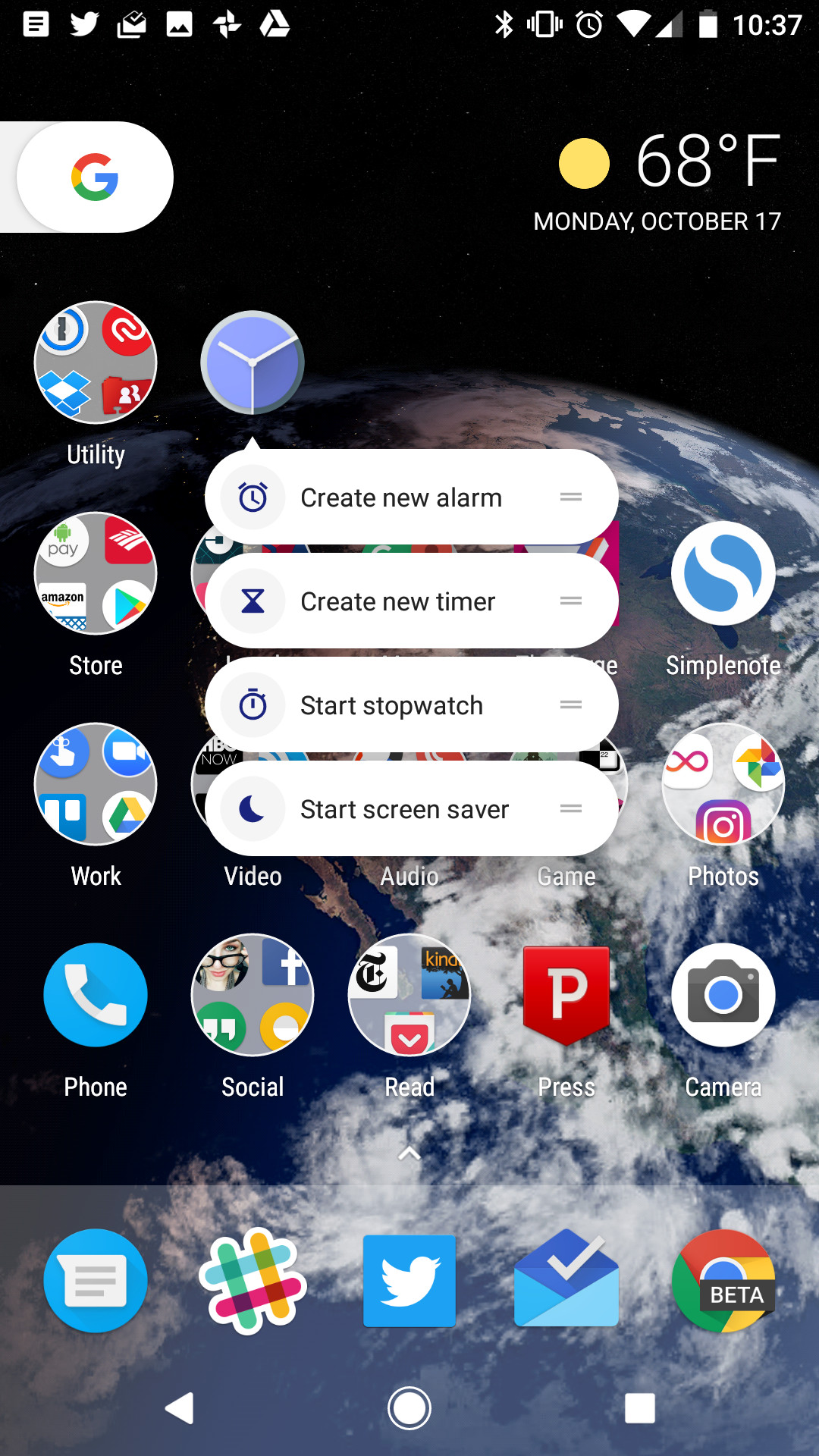A detailed and cleaned-up caption for the described image could be:

---

The image shows a dark-themed computer screen displaying various elements. In the top-right corner, the time is displayed as 10:37 AM, and indicators for a strong internet connection and a fully charged battery are visible. The screen features a Google search box, and the date and weather are shown: sunny and 68 degrees on Monday, October 17th. 

The desktop background is an aerial photograph of Earth, prominently showcasing clouds and landmasses. Various icons are present on the desktop, starting with an icon labeled "Utility." Beside it is an icon characterized by a purple cube within a circle. 

Below these icons, there are dropdown menus with options such as "Create New Alarm," "Create New Timer," "Start Stopwatch," and "Start Screensaver." Additional icons are listed beneath "Utility," including "Store" and several others partially obscured by dropdown menus. 

The remaining icons include: "Simple Note," "Think Note," "Work," "Video," "Audio," "Photos," "Phone," "Social," "Road," "Read," "Press," and "Camera," indicating a variety of applications available on the device. Along the bottom of the screen, various media site tabs are open.

---